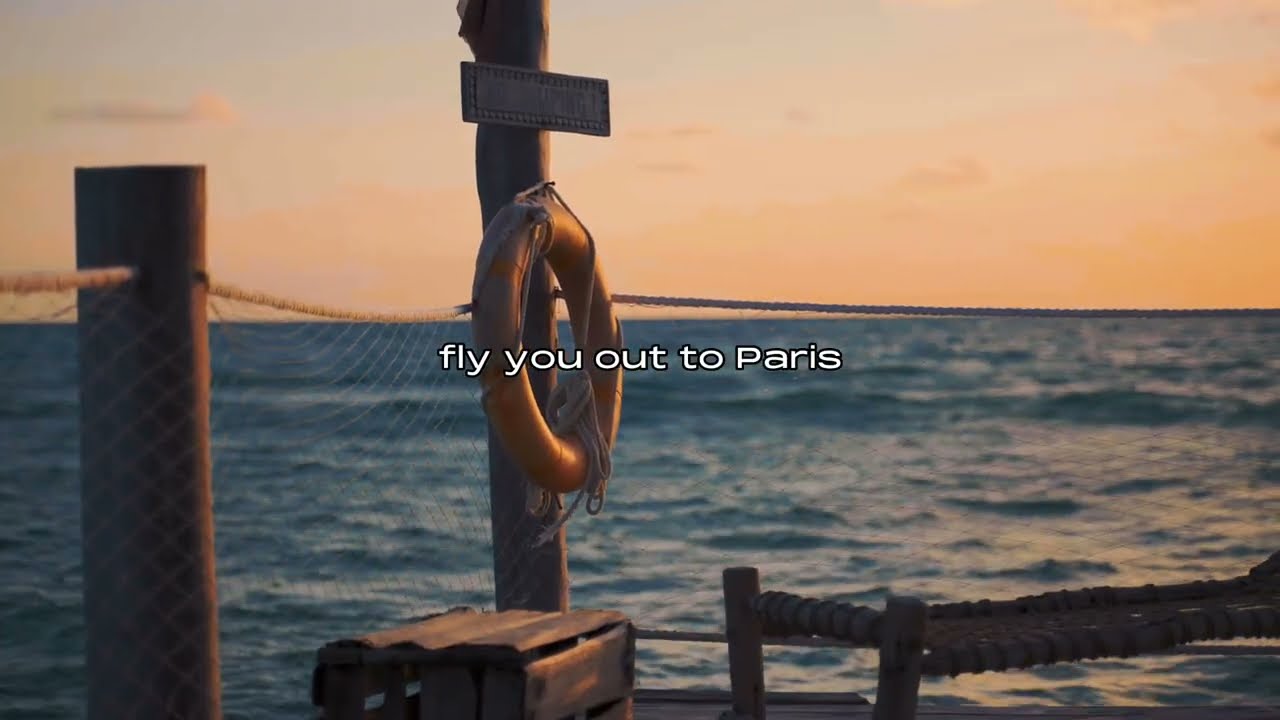The image depicts a beautifully detailed waterfront scene with a vibrant sunset casting an orange and yellow glow across the sky, suggesting it's taken during the evening hours. The background features deep blue water with visible ripples, creating a tranquil, flowing effect. In the foreground, there's a dock or raft constructed from wooden planks. Prominently, a wooden pole stands with a rectangular sign, displaying the message "Fly you out to Paris" in white text.

Attached to the pole is an orange life preserver, indicative of safety measures near water. Immediately below, a wooden box sits on the dock. There's a second wooden post to the left, connected by netting that resembles fishing nets or rope, giving a rustic maritime feel. Additionally, there are two smaller poles surrounded by gravel on the lower right side, and a structure that looks like a bed frame with woven fibers, enhancing the impression of a raft. Overall, the scene is a harmonizing blend of water, safety elements, and a picturesque, serene sunset.